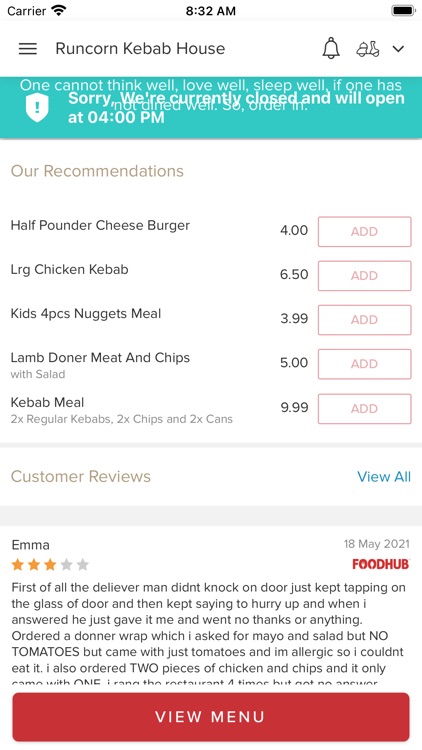The image showcases a page from a door delivery app featuring the restaurant Runcorn Kebab House. The main banner indicates, "Sorry, we're currently closed and will open at 4pm." Overlaying this banner is another text, though less bold and harder to read, stating, "One cannot think well, love well, sleep well if one has not dined well. So order in." This appears to be a social media ad text. At the bottom, there is a partially visible customer review by Emma, dated May 18, 2021. Emma gave the restaurant three stars, mentioning issues with the delivery man not following instructions and the custom order not adhering to her specifications, which is particularly concerning due to her allergies. At the top of the page, the app highlights some of the restaurant's most popular choices: a half-pounder cheeseburger, chicken kebab, kids' nuggets meal, and kebab meal.